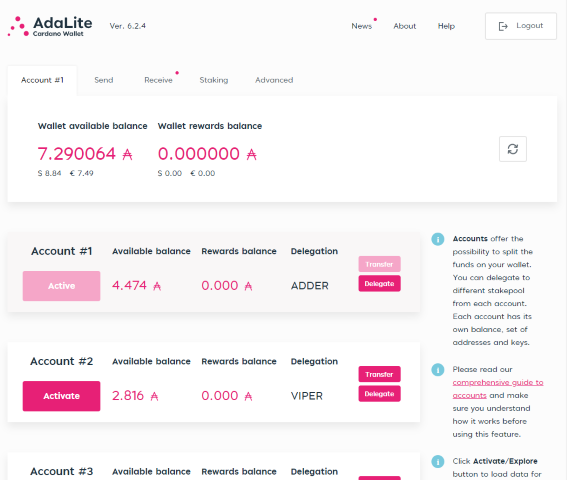The image showcases the detailed interface of the Adalight Cardona Wallet website. On the left side of the header, the website name and logo are prominently displayed, accompanied by the version number, 6.2.4. On the right side of the header, users can find a series of navigation headings such as "News," "About," "Help," and a "Logout" button.

Below the header, three main panels are organized for user interaction. The first panel lists options including "Account 1," "Send," "Receive," "Staking," and "Advanced." Currently, "Account 1" is selected, displaying the wallet's available balance and reward balance, with a refresh icon on the right for updates.

The second section further details "Account 1," showing the available balance, rewards balance, and delegation status, which is identified as "Addera." The "Active" button under "Account 1" is highlighted in light pink, indicating it is already active. Additionally, the "Delegate" button is enabled, suggesting it is clickable.

Further down, "Account 2" is listed with a status of "Activate," meaning it hasn't been activated yet. Similar to "Account 1," it also shows the available balance, rewards balance, and delegation status, which in this case is "Viper." Both the "Transfer" and "Delegate" buttons for "Account 2" are enabled.

On the far right side of the interface, there is a section of explanatory text providing information on account management, detailing processes such as activation and exploration.